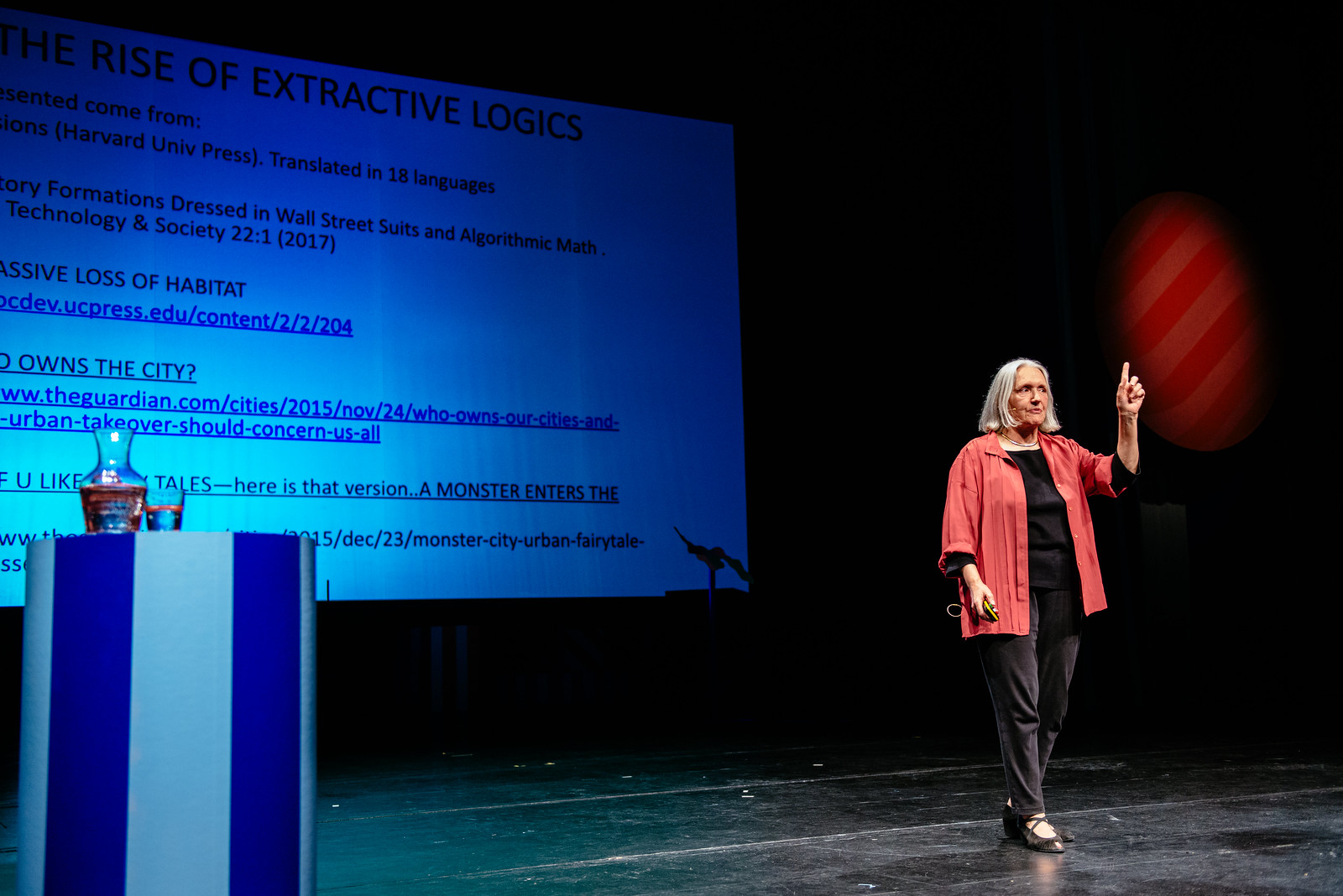This detailed landscape-oriented color photograph captures an interior view of a stage scene with a woman in her early 60s delivering a lecture. She is Caucasian, with gray, shoulder-length hair cut to her chin. She wears a long-sleeved, unbuttoned red top over a black long-sleeved shirt and black pants, paired with black shoes. 

She is standing on the right side of the stage, holding a device to change slides, and uses her left hand with her index finger raised to illustrate a point. Near her mouth is a microphone, enhancing her audibility to the audience. 

In the background, a large projection screen displays her presentation titled "The Rise of Extractive Logics." The screen features a blue background with the title in black lettering across the top and several topic points with referenced URLs below. 

To her left, in the front corner of the stage, is a multicolored podium painted with vertical stripes of light blue and dark blue, adorned with a glass and a carafe of water. The scene combines photographic realism with clear representational details, offering a comprehensive view of the lecture setting.